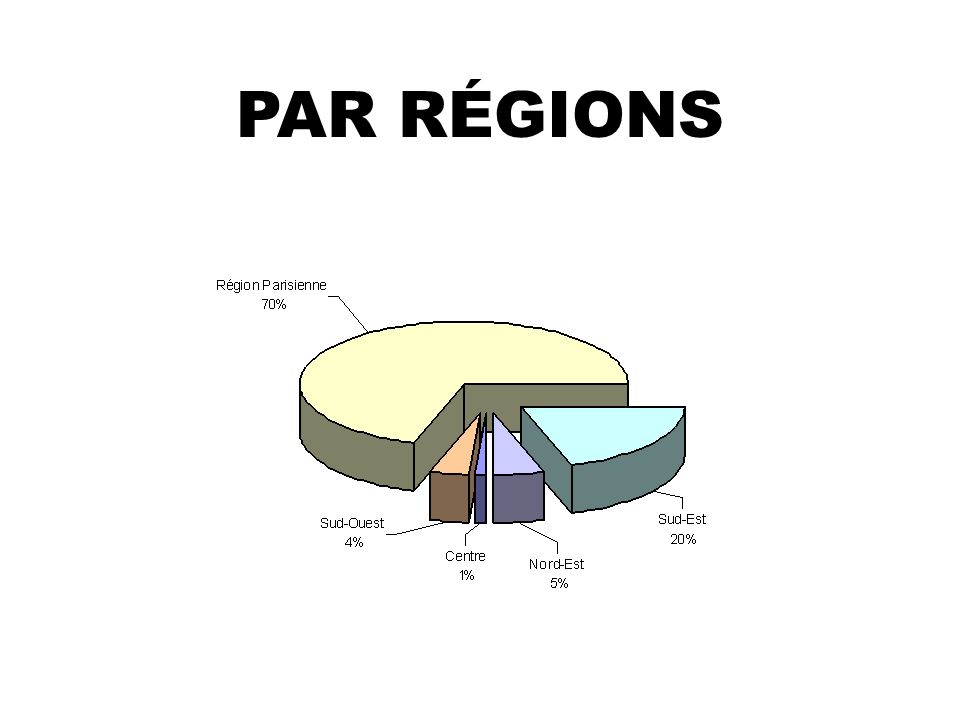The image is a detailed pie chart titled "Par Régions" (with an accent on the 'é') in a bold, blocky black font with a slight mauve shadow, giving it a 3D effect. The chart, entirely in French, represents the distribution of various regions within Paris and its suburbs. The largest section, occupying 70% of the chart, is labeled "Région Parisien" and depicted in a very pale yellow, resembling a large Pac-Man shape. Smaller sections originate from the lower right of this main portion: "Sud-Est" at 20% in a pale light green, "Nord-Est" at 5% in pale purple, "Ouest" at 4% in orange, and the "Centre" at 1% in dark purple. Additional colors present in the chart include teal, turquoise, and a sliver of blue. The background of the pie chart is white. The image seems to convey a subdivision of Paris's main region into several distinct parts, indicating a detailed focus on the spatial distribution and possibly for a business or geographical presentation.